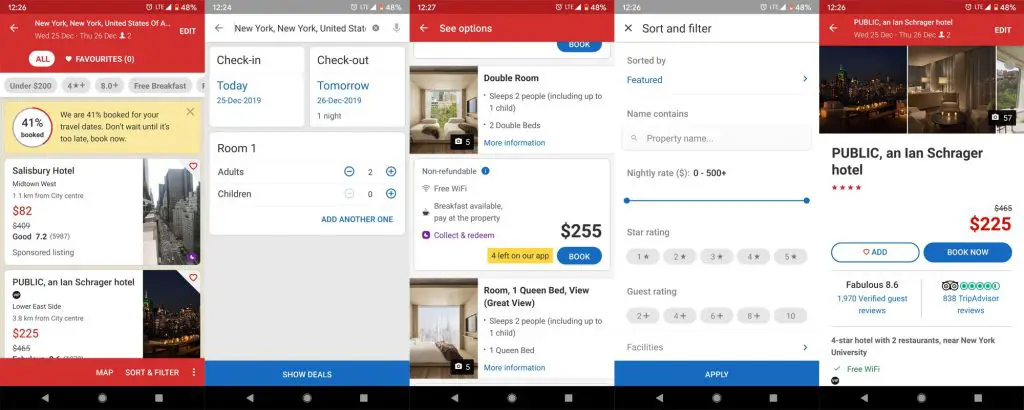The image appears to be a screenshot of a hotel booking website, specifically formatted for mobile devices. The visual is split into four sections, each capturing different stages of the booking process.

From the leftmost segment, there is a red-bordered area showcasing a list of hotels, including Salisbury Hotel, Public, and Ian Scringe Hotel. A user seems to have selected a booking option, revealing a pop-up screen to its right.

The central pop-up highlights booking details for a stay in "New York, New York, United States." The check-in date is the 25th of December, followed by a check-out on the 26th of December, 2019, indicating a one-night stay. It specifies accommodations for "Room 1" with two adults and no children. At the bottom, there is a blue "Show Details" button.

The third segment to the right features additional hotel options, including a double room priced at $255. Another pop-up screen in this section presents sorting and filtering choices, allowing users to arrange options by "Nightly Rate" (ranging from $0 to $500), "Star Rating," and "Guest Rating." At the bottom of this filter menu is a blue "Apply" button.

In the far-right section, the user appears to have selected additional hotels, Public and Ian Scringe Hotel, listed at $225 per night. This section includes an "Add" button and a blue "Book Now" button, emphasizing the booking call-to-action.